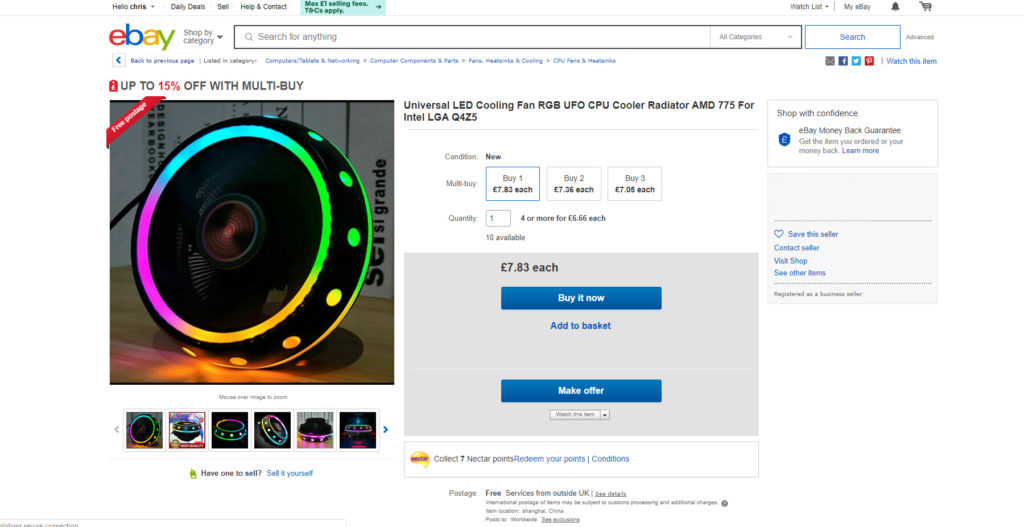**Detailed Caption**:
This image showcases an eBay listing for a "Universal LED Cooling Fan RGB UFO CPU Cooler Radiator" compatible with AMD 775 and Intel LGA 115x sockets. Priced at £17.95 each, discounts apply when purchasing multiple units: £7.30 each for 2 units, and £7.05 each for 3 or more units. The listing indicates that around 1,783 units have been sold. The displayed price is in pounds, suggesting the seller is based in Europe. The image portrays the RGB LED cooling fan, a popular accessory for enhancing the aesthetics and cooling efficiency of gaming PCs. Offers are accepted in addition to the 'Buy It Now' option, and the seller appears to have a substantial inventory. The listing also mentions discounts of up to 15% for bulk purchases. The overall presentation is geared towards tech enthusiasts looking to upgrade their computer cooling systems with visually appealing components.